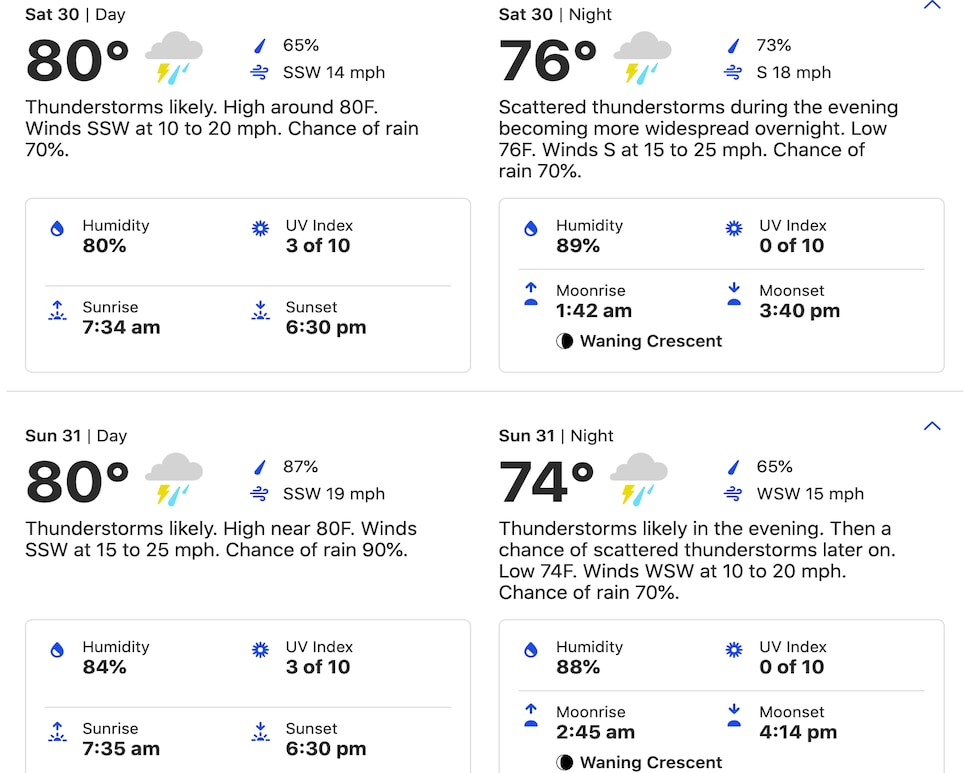A screenshot displays a variety of weather-related forecasts for Washington State University, presented on a white background. The forecasts indicate temperatures of 81°F, 76°F, and 80°F, with one showing 74% humidity. Additional metrics include the UV index, sunrise and sunset times, and wind speeds. Cloud icons signify weather conditions. There is a visible drop-down error in one of the forecasts. The top of the image is slightly cut off, making it difficult to determine the specific app being used.